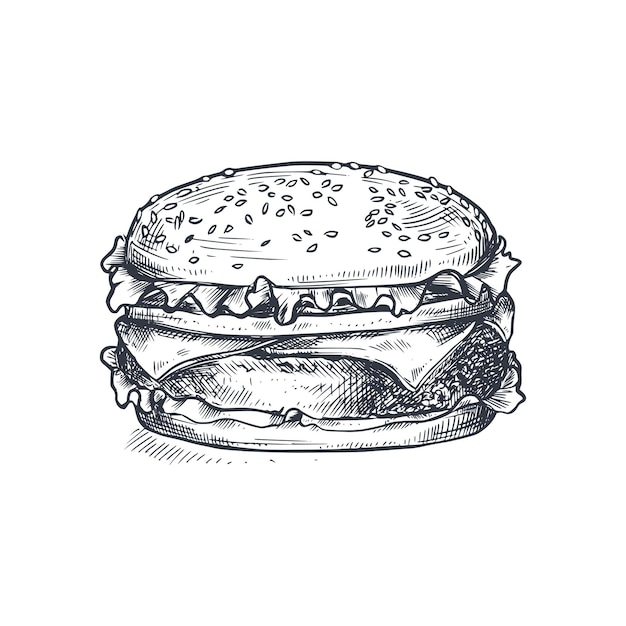This black-and-white drawing showcases a stylized and intricate depiction of a cheeseburger created using pen and ink or pencil sketch techniques. The artwork features a sesame seed top bun with seeds scattered across it. Beneath the top bun, there is a layer of lettuce followed by a slice of tomato. Below the tomato, two slices of cheese are placed on either side of a crisscrossed, line-shaded burger patty, giving the drawing depth and texture. Further down, there is another layer of lettuce and some dripping sauce visible on the left side. The bottom bun supports the entire structure of the burger. The use of horizontal and vertical lines, as well as hash marks, creates various shades and highlights, adding to the detailed and artistic presentation of the cheeseburger.